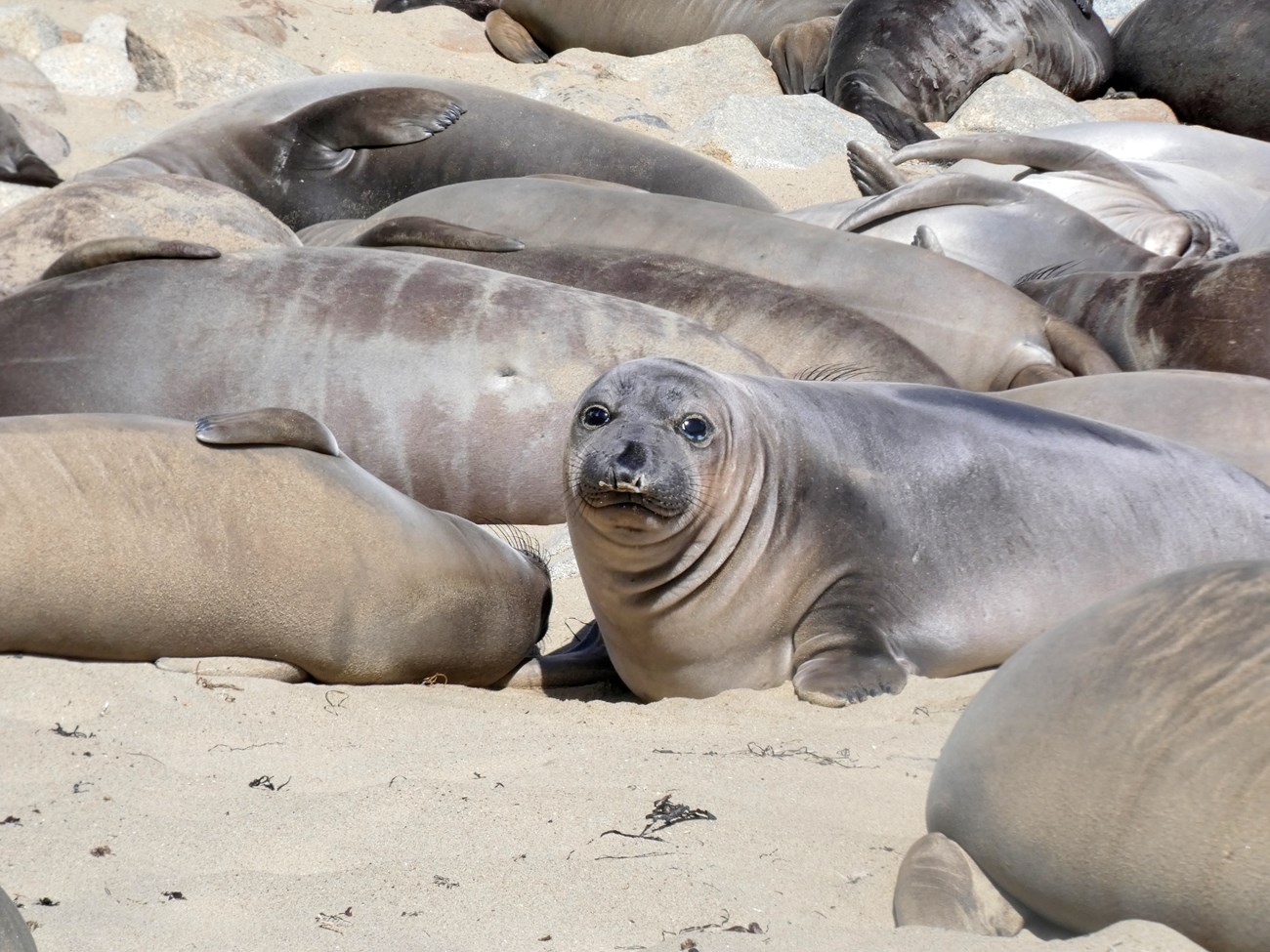A group of sea lions bask in the sun, sprawled across the sandy beach in the foreground. The sun bleaches the scene, where a dozen sea lions lie horizontally, some appearing to be asleep while others simply lounge. Among them, one sea lion stands out, lifting its wrinkled, tan chin and looking directly at the camera with big eyes, its grey body contrasting against the lighter areas on its underbelly and mouth. Scattered kelp or seaweed adds texture to the beachscape. The background features sand-colored rocks, adding a rugged frame to the sunny setting. Among the sea lions, another one is partially visible in the lower right corner, with just a hint of its body peeking into view. The serene atmosphere highlights the calm, sleepy nature of these marine animals, with the jagged edges of their flippers resting against the sand.